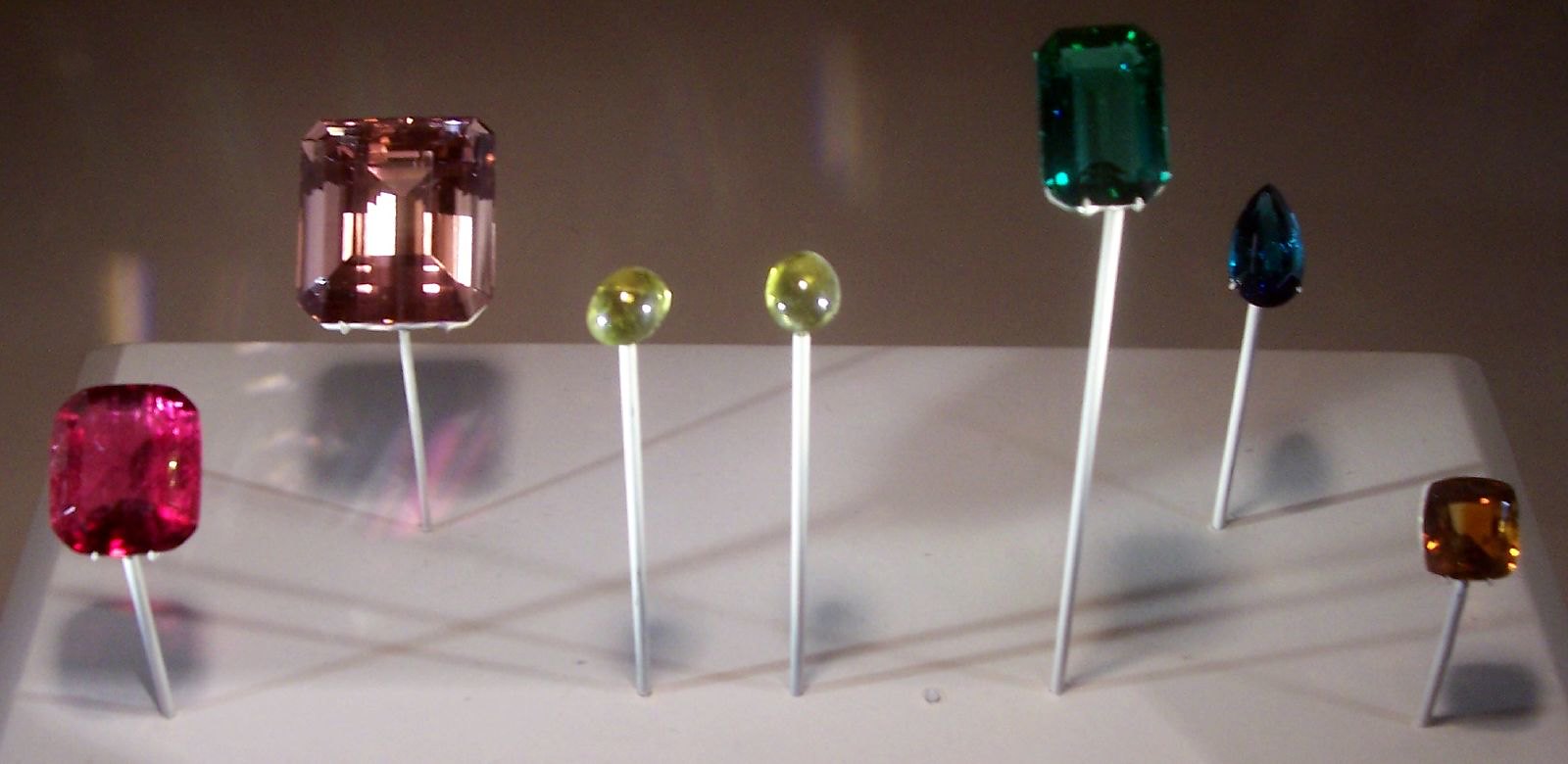The photograph captures a display of seven distinct gemstones, each meticulously mounted on small white rods, elevated above a pristine white table. The gemstones are arrayed in two rows against a brown backdrop. Starting from the bottom left in the front row, there is a square pinkish-red gem that catches numerous shadows and shines brightly, resembling a ruby. Adjacent to it in the middle are two light green circular gems with slight imperfections, akin to green grapes. To their right is a deep forest green rectangular gem, likely an emerald, reflecting a significant amount of light. Further right, almost at the bottom right corner, is a small square orange gemstone.

In the back row from left to right, there is a larger square brown gem that reflects rectangular lights vividly. Positioned further back on the far right is a bright blue teardrop-shaped gem, possibly a sapphire. Each gem is made to stand out, mounted on the slender white rods, creating an organized yet visually captivating arrangement inside what appears to be a display case.